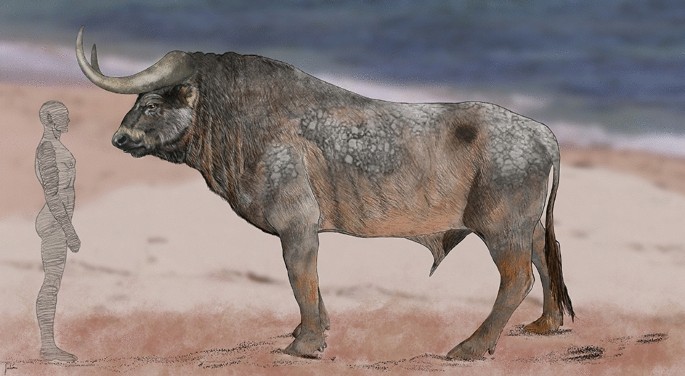In the image, a meticulously detailed and realistic depiction of a large bull faces a sketched silhouette of a man. The bull, with its impressive stature, stands on a sandy beach with visible footprints, set against a backdrop of the blurred blue ocean and whitecaps. The bull's coat is a mix of brown, black, and gray fur, with rough, scaly spots visible on its upper left shoulder, side, and hindquarters. Its long, hairless tail ends in a tuft like a ponytail. The bull's formidable horns, which curve upward from its head, add to its majestic appearance. The sketched man, rendered with pencil lines from head to toe, stands nude in profile, almost reaching the bull's eye level but dwarfed by the animal's larger size. The scene creates a stark contrast between the detailed, life-like bull and the simplistic, gray silhouette of the man, capturing a moment of silent confrontation on the light tan sands of the beach.